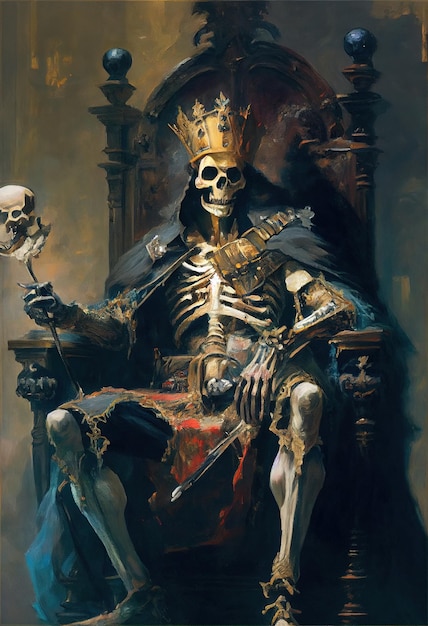This image is a meticulously detailed illustration of a skeleton king seated on an ornate, dark brown wooden throne. The throne's design features two posts on either side, each topped with a small sphere, and its high back is rounded at the top. The background is a wall shaded in dark tones of orange, brown, green, and yellow.

The skeleton king, adorned in tattered and dirty attire, wears a tall crown that alternates between descriptions as orange and gold. He is draped in a black, decaying cape and what appears to be a tattered kilt. His left elbow rests on one arm of the throne, while his right hand grips a staff or spear topped with a skull. A black feather adorns the throne, adding to its regal yet eerie appearance.